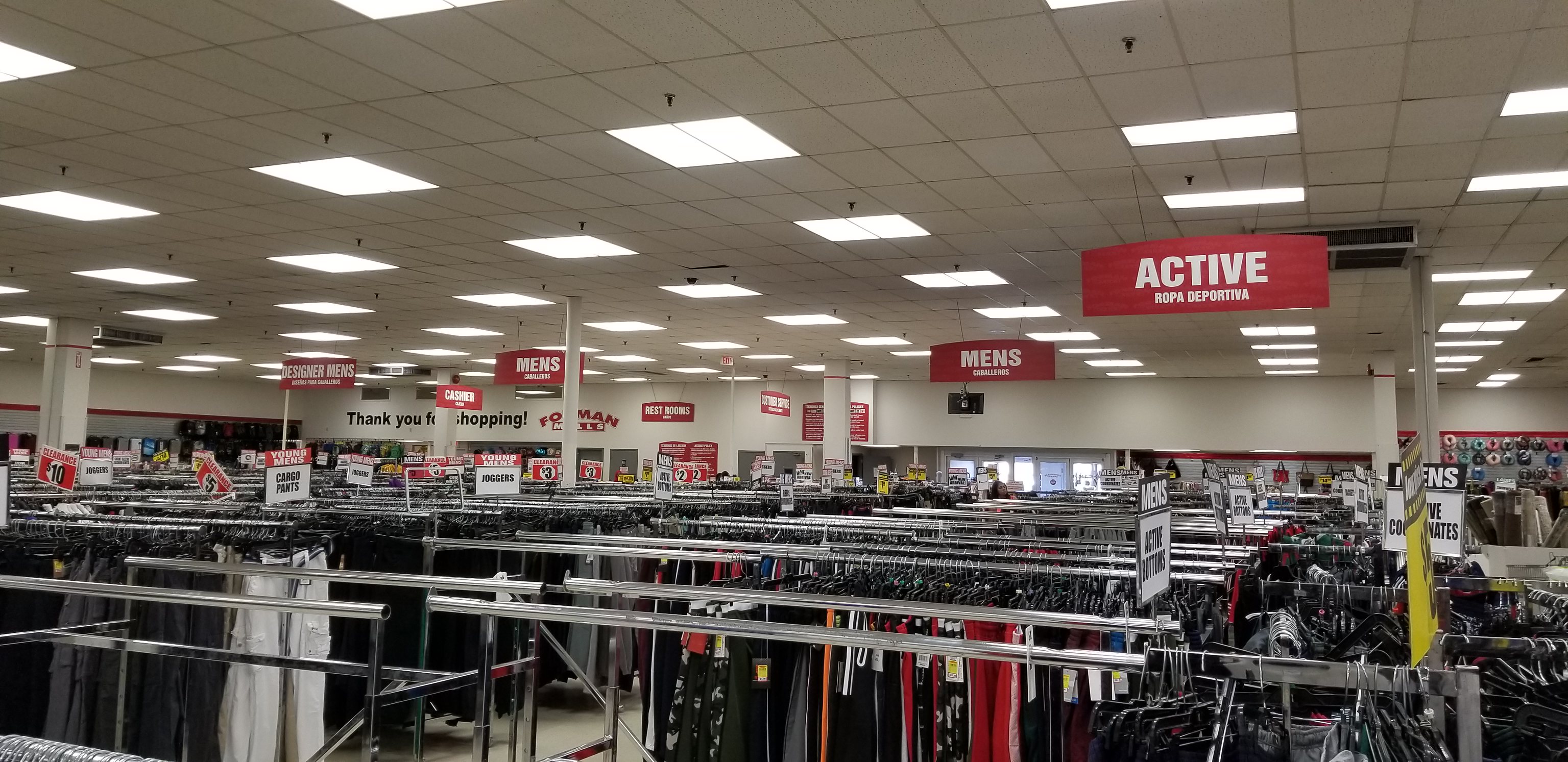This photograph captures the interior of a clothing department store. Rows of metal racks filled with a diverse array of clothing items such as pants, shirts, sweaters, and hoodies populate the space. Near the front, a few racks stand empty. Overhead, red signs with white text designate different sections, including 'Active' and 'Men's,' while additional signs on the left remain indistinct. Text on the back wall, partially obscured by structural support pillars, reads "Thank you for shopping." In the background, large glass doors suggest entrance and exit points, likely consisting of two sets of sliding doors. Overall, the store appears spacious and well-organized, offering a variety of clothing options for shoppers.